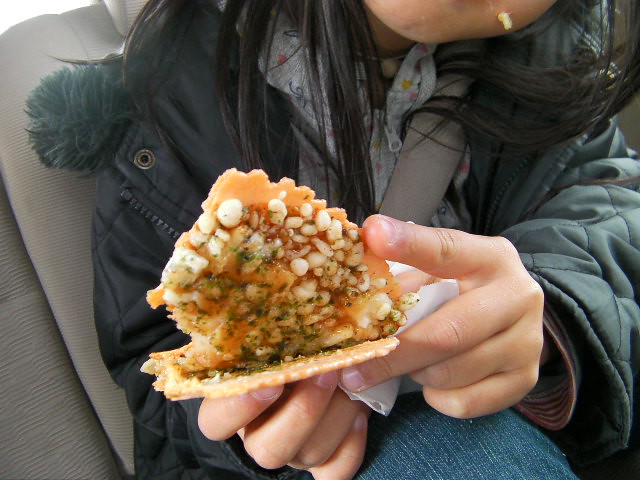A person with medium-toned skin is seated in a car, which has a light gray interior and a gray seatbelt fastened across their chest. They are wearing blue jeans and a dark, parka-like, black or dark green coat with a faux fur-trimmed hood. Beneath the coat, a multicolored pattern can be seen on their shirt. Their long, straight black hair drapes over their chest as they hold a piece of food in their left hand, presenting it towards the camera. The food appears to be a type of flatbread or pastry, torn open to reveal its contents which include possible red sauce, cheese, beans, rice, onions, and spices. The bright sunlight highlights the scene, suggesting a daytime setting. The person’s face is partially visible, showing just the lower part including their chin and some of their cheek.